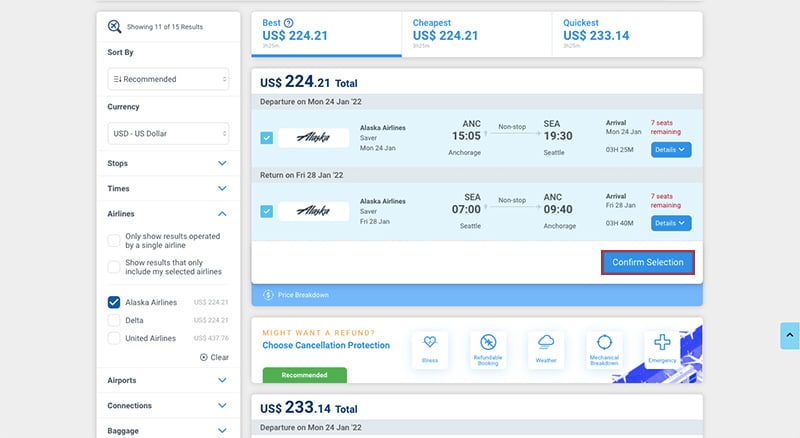Screenshot of a flight booking section on a travel website, presenting various details and options for selecting a flight. The left-hand side features a large filter box indicating "Showing 11 of 15 results". Several filtering options such as "Sort by" which is currently set to "Recommended", and "Currency" set to "USD" (United States Dollar), are visible. Additional filter categories include "Stops", "Times", and "Airlines". The airlines filter is open, showing options for Alaska Airlines (checked), Delta, and United Airlines, with choices to show results operated by a single airline or include only selected airlines. Closed filter options mentioned are "Airports", "Connections", and "Baggage".

On the right-hand side, the cheapest fare highlighted in blue is priced at $224.21 for an Alaska Airlines flight from Anchorage (ANC) to Seattle (CSEA), departing at 15:05 and arriving at 19:30 with 7 seats available. This flight is for a trip departing on Monday, January 24, 2022, and returning on Friday, January 28, 2022. The return flight departs at 07:00 and arrives back at 09:40, with 7 seats remaining. 

Beneath this, there is a red "Confirm Selection" button framed in a red box for easy selection. Another flight option priced at $233.14 is partially visible below but cut off so detailed information is not displayed.